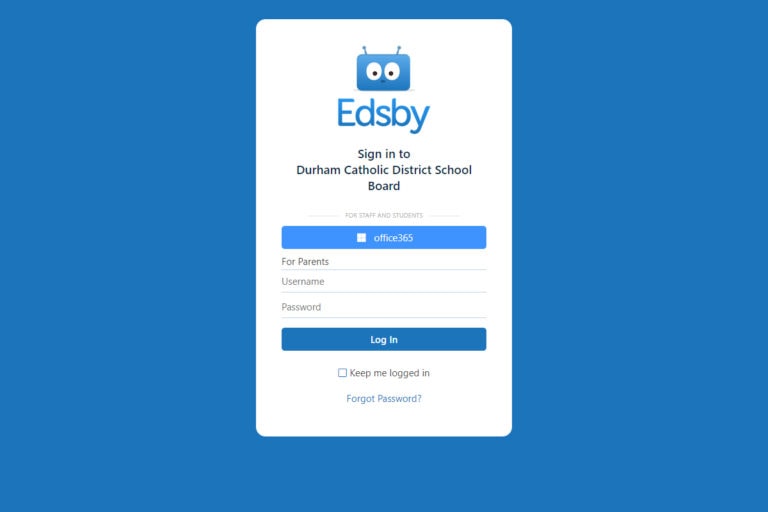In this image, we see a detailed screenshot set against a blue background. The primary focus is a white rectangular section positioned horizontally within the blue frame. At the top of this section is an icon depicting a blue robot's head, complete with two antennas, googly eyes, and a straight-line mouth. Directly below the icon, blue text spells out "Edsbee."

Underneath "Edsbee," there is black text that states "Sign in to Durham Catholic District School Board." Below this heading, you will find a blue action button labeled "For Staff and Students, Office 365."

The lower portion of the white rectangle contains a form with three distinct lines: the first line is designated for parents, the second line prompts for a username, and the third line requests a password. Following the form, there is a dark blue action button that reads "Log In."

Near the bottom of this section, there is small black text on the white background that says "Keep me logged in," and, directly below that, blue text that provides a link reading "Forgot Password."

Overall, the image is a login page interface for the Durham Catholic District School Board, clearly guiding users through the process of signing in and providing help in case they forget their password.